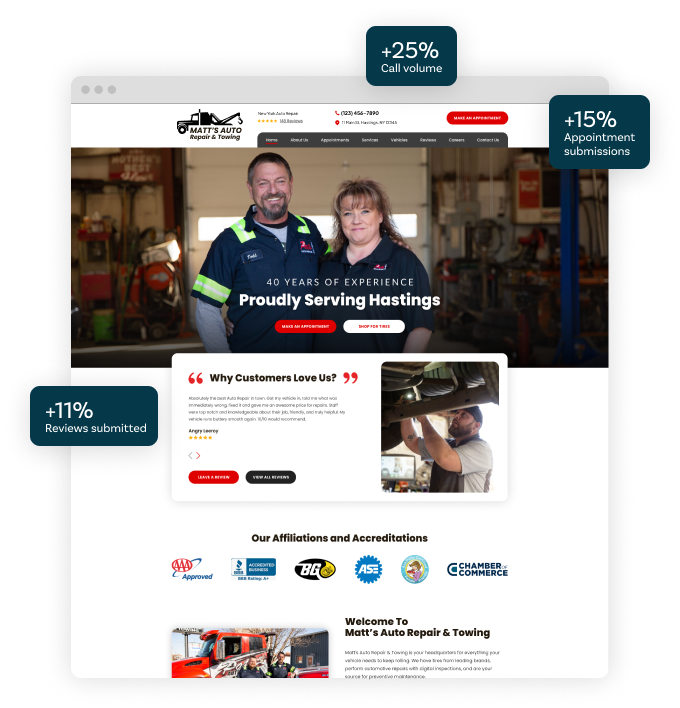This is the homepage for Matt's Auto, featuring a sleek and professional design that immediately conveys the business's expertise and customer focus. At the top, a white banner prominently displays a black truck logo with bold black text reading "Matt's Auto Repair and Towing," accompanied by the central placement of the business's phone number. To the far right, a noticeable pop-up proudly states a "+15% increase in appointment submissions," hinting at growing customer engagement. Just above it, another pop-up in blue with white text highlights a "+25% call volume increase," showcasing enhanced communication.

Central to the page is an image of a smiling Caucasian middle-aged couple, exuding warmth and reliability. The man, with short dark brown hair, a close-cut beard, and hints of gray, wears a dark blue shirt. Beside him, a woman with light brown hair and bangs also wears a dark blue shirt, mirroring professionalism and unity. Superimposed on this image in bold white text are the words "40 years of experience," followed by "Proudly serving Hastings" directly underneath.

Below this central image, two interactive click bubbles stand out: the first being red with white text, and the second white with red text, designed to engage visitors further. A text rectangle beneath these bubbles features black text that reads "Why customers love us," introducing a customer review section. Adjacent to this, a photograph captures a mechanic diligently working on the underside of a car, illustrating the hands-on expertise and care provided by Matt's Auto.

The homepage concludes with a section labeled "Our affiliations and accreditations," where respected logos of AAA Approved, Better Business Bureau, BGASE, and the Chamber of Commerce are displayed. These affiliations underscore the trustworthiness and recognized quality of Matt's Auto services.